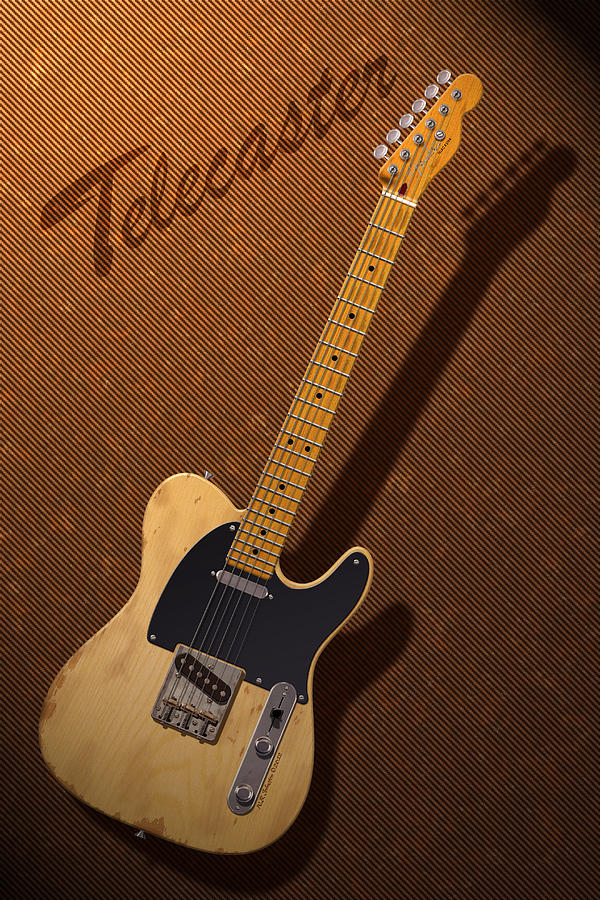The rectangular photograph features a prominently placed wooden electric guitar, specifically a Telecaster, with the word "Telecaster" in handwritten brown text overlaid in the top left corner. The guitar is strikingly detailed, with a wood grain finish and a distinct black plate on the body where one would typically strum. The instrument spans diagonally from the bottom left to the upper right, with the base towards the bottom left corner. It also has a worn look in some areas and includes metallic elements such as knobs and the metal plate holding the strings. The background is textured, resembling a cardboard wall in varying shades of dark to light brown, giving a sense of depth with a clear shadow of the guitar cast onto it. The image is highlighted by a light source in the top left-hand corner, adding a dramatic illumination to the scene. This photograph could very well be part of an advertisement for musical instruments, given its stylish presentation and clear emphasis on the guitar.